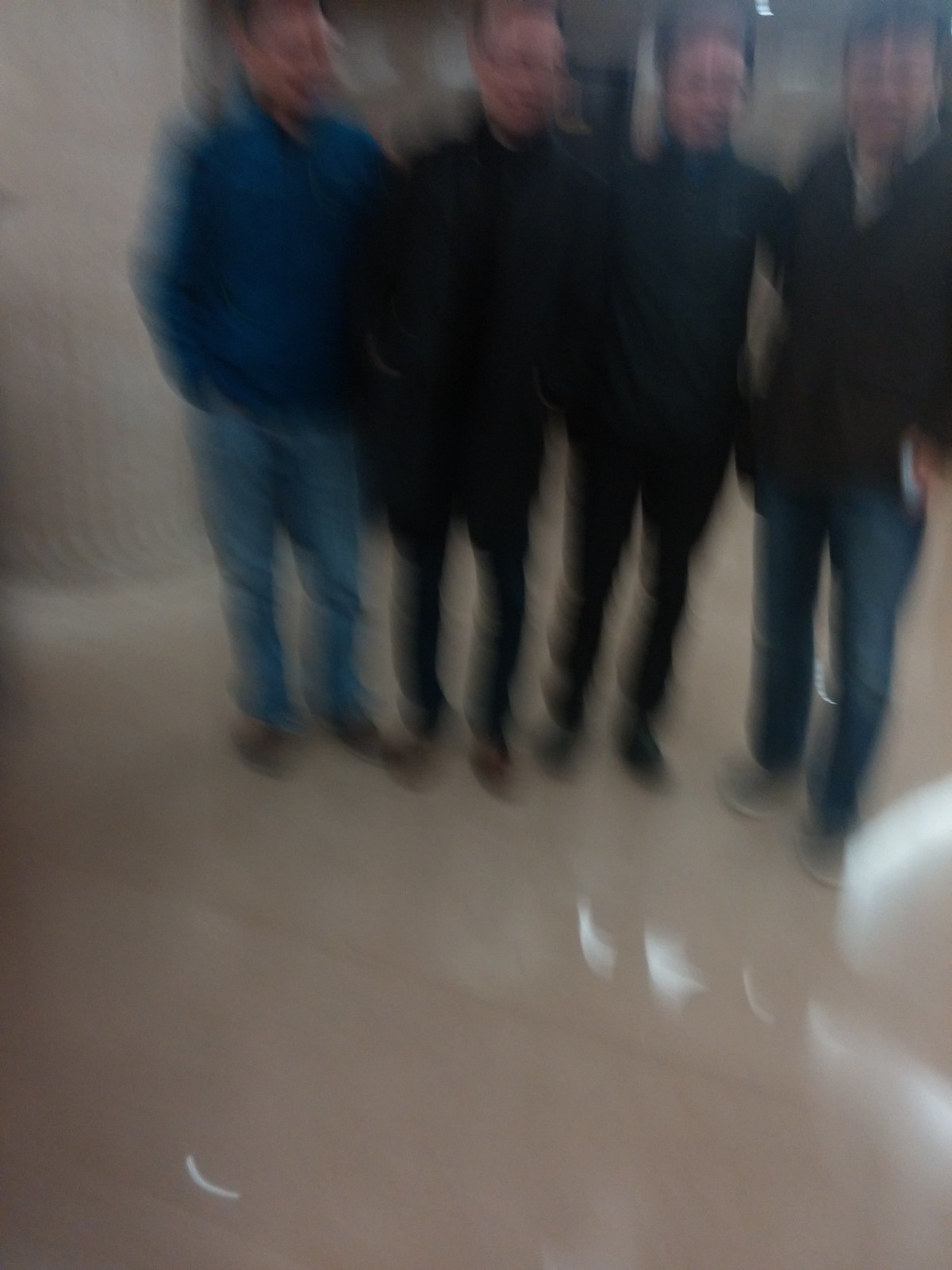In this blurry photograph, we see four men standing side-by-side inside what appears to be the lobby of an office building or hotel. The background features what seem to be doors or elevator doors. The highly polished, cream-colored stone floor—suggesting marble—reflects the bright lighting of the space. All four men are facing the camera, smiling, with receding hairlines and wearing glasses. Their attire includes casual outfits: the man on the left dons a blue jacket and blue jeans, the second and third men are both dressed in black jackets and black pants, and the fourth man sports a brown jacket and blue jeans. They all appear to be wearing either tennis shoes or dress shoes. Despite the photo's significant blurriness, the men's cheerful expressions and casual stance with hands in pockets suggest a moment of camaraderie, albeit captured by an unskilled photographer.